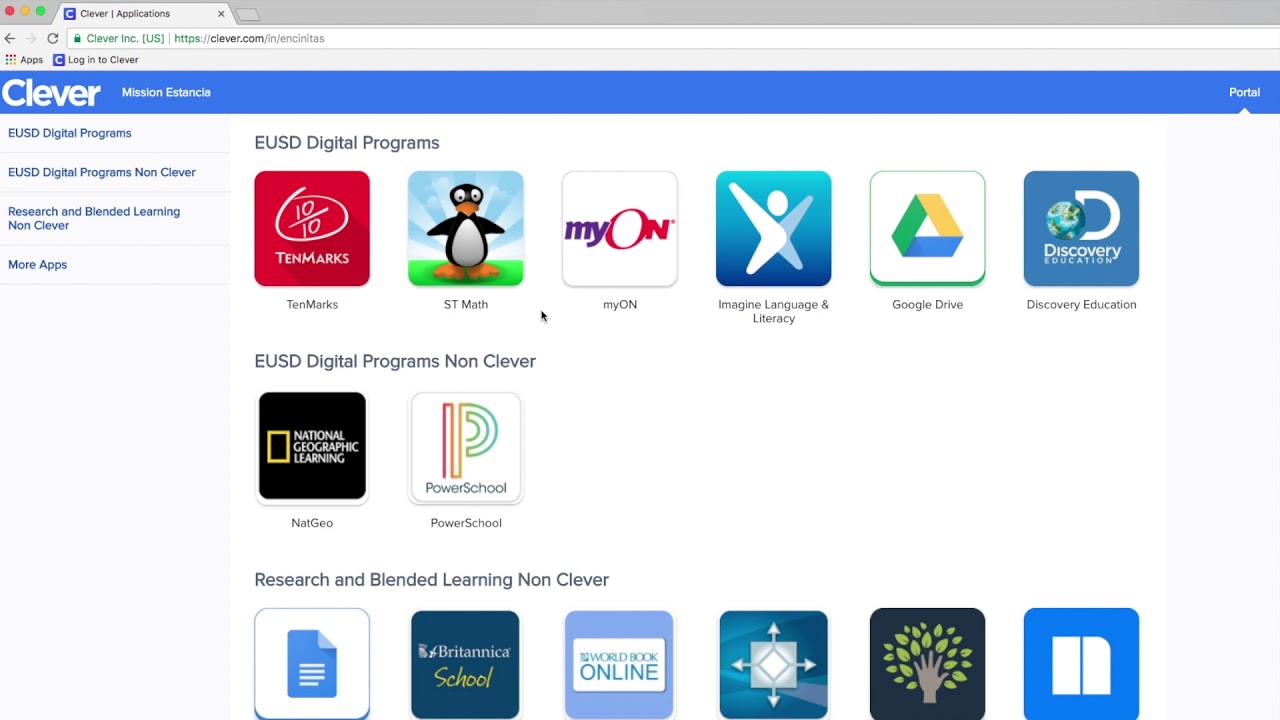The image is a screenshot of a website displayed in the Safari browser. In the top left-hand corner of the screen, the Safari browser interface is visible, featuring the three standard control buttons: a red circle for closing, a yellow circle for minimizing, and a green circle for maximizing the window. Only one tab is open, labeled "Clever Applications."

Below the tab bar, there is a search bar displaying the URL "https://clever.com" and the text "Clever Inc. USA." The remaining URL details are partially obscured due to small gray font. Beneath this, a blue banner spans the width of the webpage. In white text, it reads "Clever Mission Estancia," and in the upper right-hand corner of the banner, the word "Portal" is displayed.

On the left-hand side of the website, a side navigation menu lists several tabs: "EUSD Digital Programs," "EUSD Digital Programs Non-Clever," "Research and Blend Learning Non-Clever," and "More Apps."

The main content area of the website showcases a variety of educational applications, arranged in three rows against a white background. Each application is represented by its icon and name:
- "10marks," featuring a red icon.
- "SDMarch," depicted with a penguin icon.
- "MyOn," identified by the simple text "MyOn."
- "Imagine Language and Literacy," displaying a character on a blue background.
- "Google Drive," represented by the distinctive Google Drive logo.
- "Discovery Education," marked by the Discovery Channel logo.
- "NatGeo," labeled as "Natural Geographic Learning" with an orange square on a black background for its logo.
- "PowerSchool," identified by a rainbow-colored "P" logo.